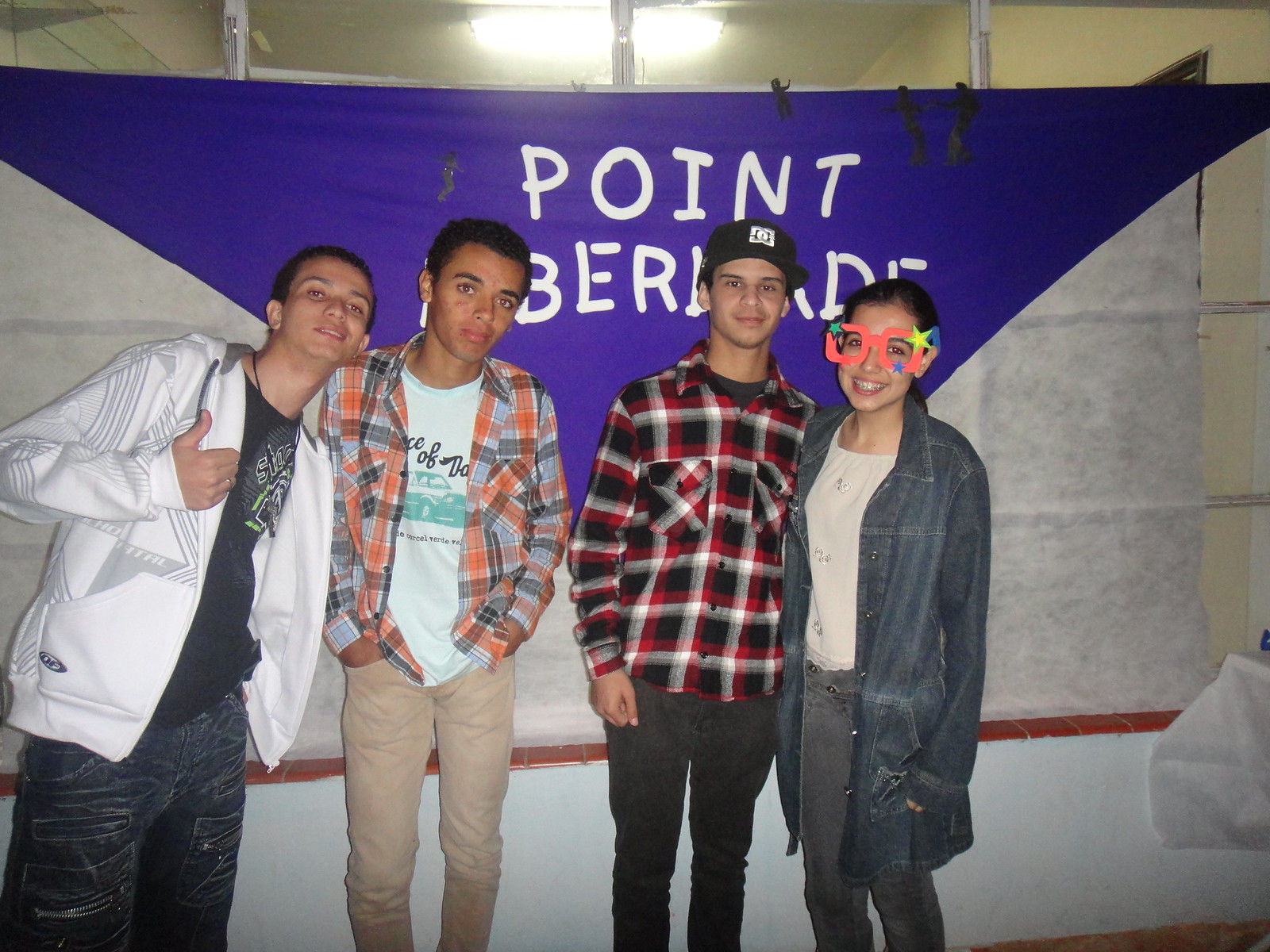The image depicts four young individuals, likely middle or high school students, standing in front of a grey stone wall. From left to right: the first young man is wearing a white hoodie over a black t-shirt with blue jeans and is smiling at the camera while leaning slightly inward. Next to him, the second young man dons an orange, grey, and white plaid button-down shirt over a white undershirt and tan pants. The third young man sports a black hat, a red, black, and white plaid button-down shirt, and black jeans. The young woman on the far right is wearing bright orange glasses with a blue and green star design, a white blouse under a long denim jacket, and grey jeans. Behind them, partially obscured by the group, is a blue flag with white text that reads "POINT," and a partially visible second word. The setting suggests a casual, possibly school-related environment.